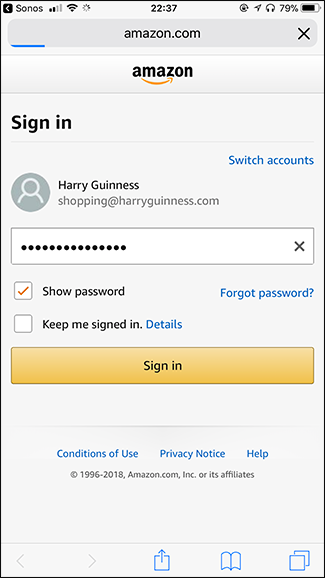This screenshot from a cell phone showcases the Amazon sign-in screen. At the top left, the provider "Sonos" is displayed, along with four bars indicating strong cell signal. Additionally, a Wi-Fi icon is present, and a loading icon suggests ongoing data transfer. In the center, the time is displayed in 24-hour/military format. On the right, various icons show a battery level of 79%, active headphones/earphones connection, location services being enabled, and the screen rotation lock being active.

Directly below the status bar, the browser search line reads "Amazon.com," partially loaded as indicated by a blue progress bar beneath it. The Amazon logo is prominently featured underneath the search line. The section beneath the logo prompts the user to sign in, displaying the name and email address "HarryGuinnessShopping at HarryGuinness.com." The password field is hidden by dots, with the option to show the password available but not selected. An orange "Sign-In" button is positioned below the password field.

The layout and elements suggest that this interaction is taking place through a mobile browser rather than the Amazon app.